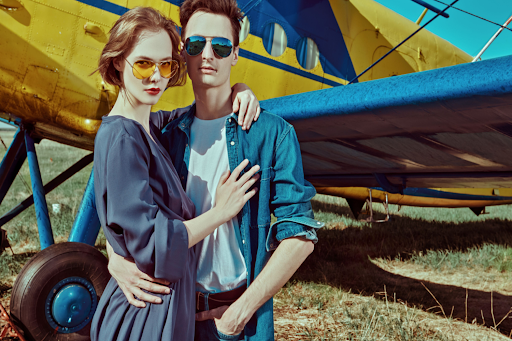In this sepia-toned photograph, a young couple, likely in their early 30s, stands closely embraced in a grassy field, gazing seriously at the camera. The woman, positioned to the left, wears a dark blue dress and yellow-tinted sunglasses. She has short hair that appears to be either red or light brown. Her left arm is draped around the man's neck, while her right hand rests on his chest. The man sports a jean jacket over a white undershirt and jeans, with aviator sunglasses shielding his eyes. His left hand is casually tucked into his pocket. Behind them, partially visible, is a classic small airplane with a yellow body and blue wings, decals, and wheels. This private aircraft, reminiscent of a vintage model with a propeller, adds an adventurous backdrop to the intimate scene.